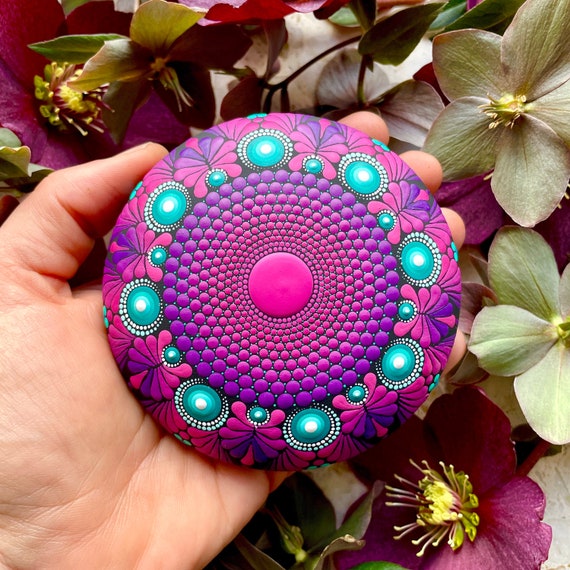In the image, a man's hand, prominently displaying the palm, holds a decorative clay disc. This circular art piece draws attention with its vibrant colors and intricate design. The centerpiece is a large pink circle, surrounded by individual drops of pink, purple, and dark purple paint, forming a mandala-like pattern that radiates outwards. As the circles expand towards the edge, they transition into larger blue, teal, and white dots, interspersed with tiny white specks. Between these larger circles are detailed flower designs, enhancing the visual complexity. The disc, possibly painted on stone, appears about the size of a drink coaster. The background is filled with dark purple and green flowers, which contrast beautifully with the hand and disc, set against what seems to be a bush with green and yellow foliage.